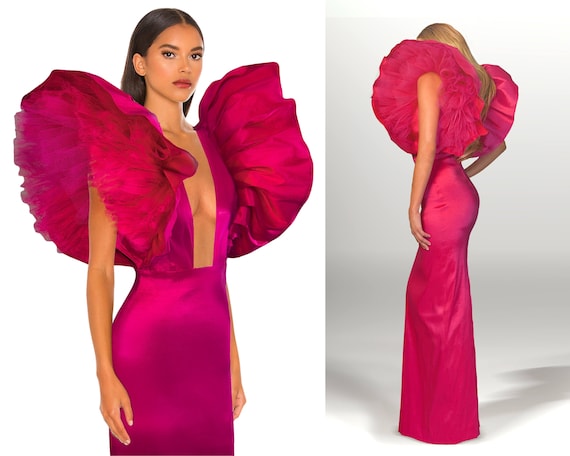The image comprises two juxtaposed photographs showcasing a striking fuchsia pink dress with both front and back views. The left photo features a model with darker skin and straight, dark brown hair slicked back, parted down the middle. She dons a bright fuchsia, tight-fitting, floor-length gown with a dramatic deep rectangular cut out in the front, exposing a center cleavage down to her navel. This gown is adorned with enormous, voluminous, poofy sleeves, richly textured and likely supported by tulle to maintain their exaggerated form. The model stands with her arms down by her sides, facing the camera directly, her expression neutral as she showcases the dress’s intricate details.

In contrast, the right photo presents a back view of the same dress, worn by a second model with long, blonde hair cascading down her back. This angle emphasizes the gown's form-fitting silhouette and the massive pink sleeves from a different perspective. The background on the left is darker, highlighting the visual details more starkly, while the right background is lighter, casting shadows that accentuate the dress's texture and the models' differing hair colors and styles. The overall composition vividly captures the dress’s bold design and lavish ornamentation from multiple angles.